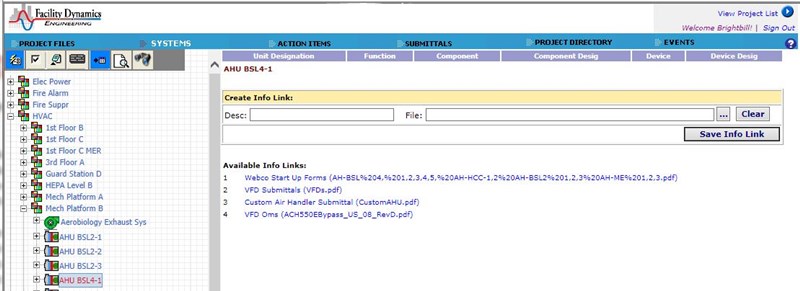The top section of the image features a white and black background with "Facility Dynamics" written on the left-hand side. This appears to be a message engine, displaying a small and blurry "S." On the right side is a gray rectangle with "View Project Lists" written in purple. Adjacent to this is a blue circle containing a white triangle.

Beneath this section, the text "Welcome, Bright Bill" is displayed in a different shade of purple, accompanied by "Sign Out" in darker purple. A horizontal line, resembling a tail border, divides the sections, bearing the label "Project Files" in white, with "system" written below in black. This is followed by additional headings in black: "Action Items," "Submittals," "Submittals" (repeated), "Project Directory," and "Events." 

A purple border runs across the next section, where the text "Unit Destination Functions" appears in white. Below this are labels such as "Component," "Component Desync," "Device," and "Device Desync." 

The background now turns white with "A-H-U-B-S-L 4-1" written in red. A yellow border follows, marked with "Create Info Link" and "D-E-S-C..." which is an empty input field. Another input field follows, labeled "File...."

Within a gray rectangle, the word "Clear" is written in purple, and another gray rectangle contains "Save Info Link" in purple. Below this, "Available Links" appears in black, followed by various labeled links in purple: "Webcoast Starter Forms," "V-F-D Submittals," "Custom Air Handler Submittal," and "V-F-D-O-M-S." 

On the other side, there are multiple labels in blue and black colors, such as "Elect Power," "Fire Alarm," "Fire Super," "A-Havoc," "First Floor B," "First Floor C," "First Floor C-M-E-R," "Third Floor A," "Guard Station D," "Headboard Level B," "MEC Platform A," "MEC Platform B," and "Chabrol Biology Exhaust." It repeats "A-H-U-B-S-L 2-1," with variations ending in "-2," "-3," and another "4-1," appearing in red with a bluish border.